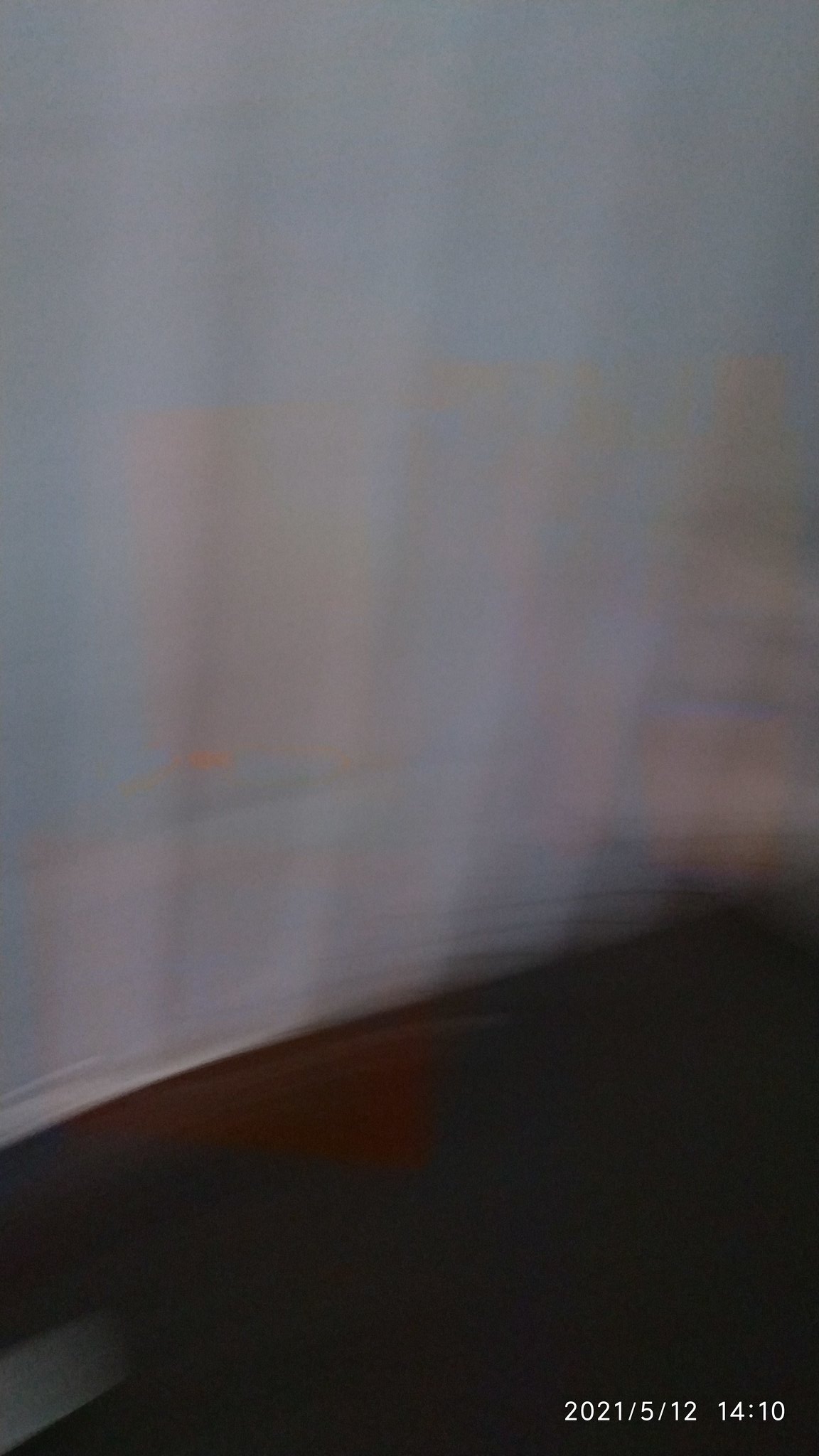The image appears to be a blurry photograph of a wall and a floor. The top portion of the image is mostly a white color with ridges, possibly resembling trim or molding, transitioning into a bluish or light blue wall that may have indistinguishable images due to the blur. The bottom third of the image is notably darker, potentially depicting a floor or a shadowed section, with an orange smudge or triangular blur that might be a reflection or focusing error. In the bottom right corner, the image displays a date, "2021/5/12," and a timestamp, "14:10." Additionally, there's a minor white blur in the bottom left corner.